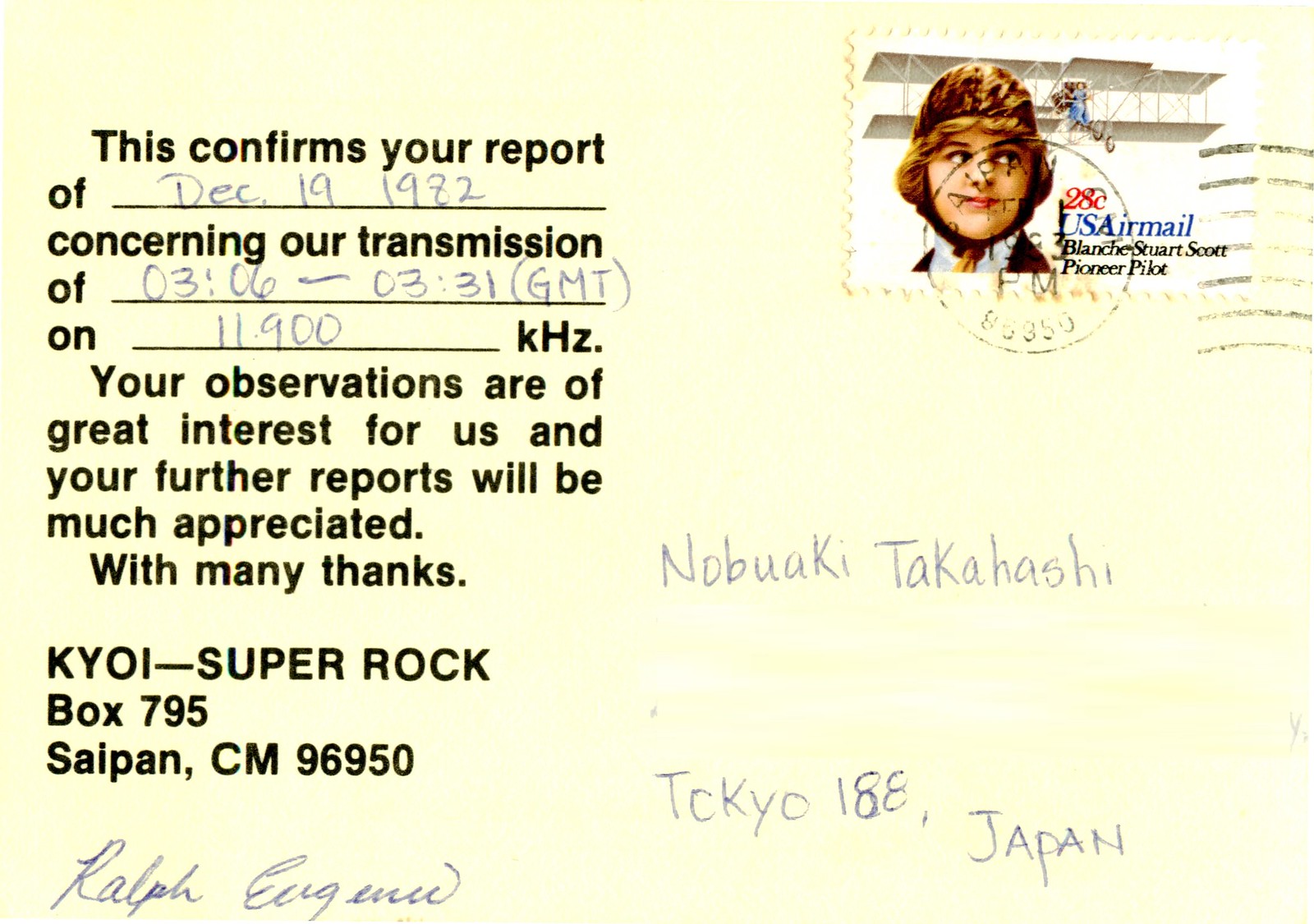The image depicts a vintage postcard with a distinct airmail stamp positioned in the top right corner. The stamp features an image of Blanche Stuart Scott, draped in a scarf and with an airplane in the background, reading "28C US Air Mail Blanche Stuart Scott, Pioneer Pilot." The postcard itself is off-white, possibly yellowed with age. On the left side of the postcard, a meticulously penned letter confirms a report dated December 19, 1982, referencing a transmission from 0306 to 0331 GMT on the frequency 11900 kHz. The text appreciates the observations and expresses eagerness for further reports, signed with gratitude by KYOI, Super Rock, Box 795, Saipan, CM96950. Additionally, the recipient’s name, Nobuaki Takahashi from Tokyo 188, Japan, is written in pen on the right side. A signature by Ralph Eugene appears at the bottom left corner of the postcard, completing this detailed correspondence artifact.